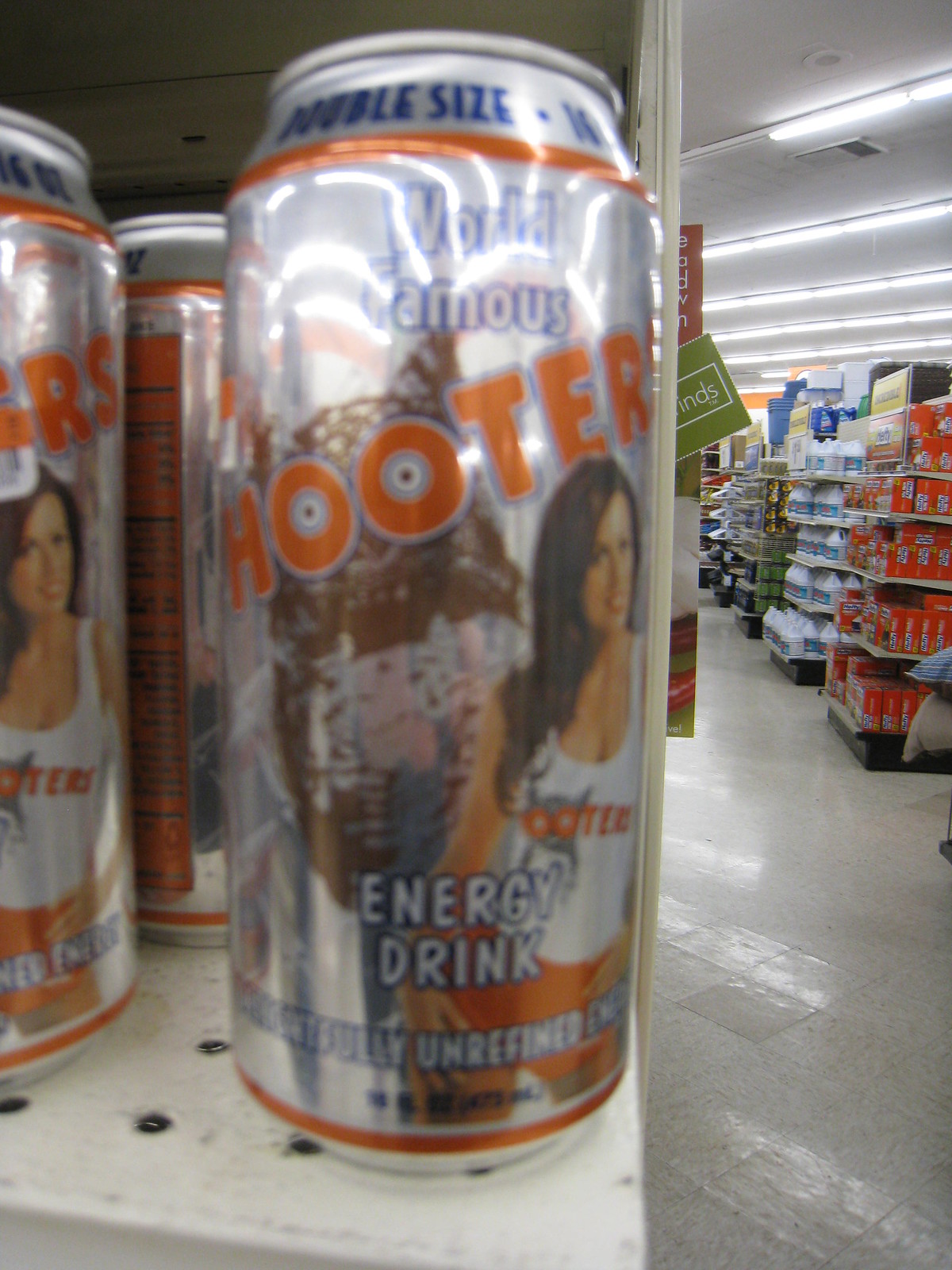This image appears to have been taken inside a store, as evidenced by the fluorescent lighting overhead and the off-white, somewhat dingy-looking tiled floor. Dominating the foreground is a silver can adorned with various colors, including navy, red, orange, white, and brown. At the top of the can, the words "DOUBLE SIZE" are emblazoned in navy font, accompanied by the phrases "world famous" in white font and "Hooter" in orange font. A detailed image of a brown owl serves as the backdrop for these texts.

Additionally, the can features an image of a model dressed in a quintessential Hooter's uniform consisting of a white tank top and orange shorts. The model is depicted with brown hair. Near the bottom of the can, the words "energy drink" are printed in white font. The Hooter's can is placed on a white metal shelf, providing a stark contrast against its vibrant packaging.